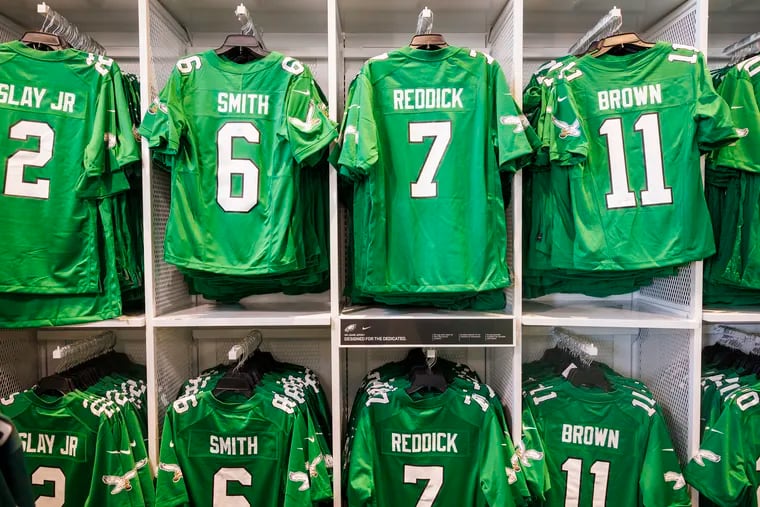This full-color, square photograph, taken indoors for display purposes, features a well-organized row of green football jerseys with white numbers and lettering, presumably in a team store or sporting goods store for the Philadelphia Eagles. The image showcases a set of ten white wooden cubbies—five on the top row and five on the bottom—each containing individually hung jerseys.

On the top row, starting from the left, is:
1. A jersey for Darius Slay Jr. with the number 2.
2. A jersey for Devontae Smith with the number 6.
3. A jersey for Haason Reddick with the number 7.
4. A jersey for A.J. Brown with the number 11.
5. Another jersey that is partially cut off and indistinguishable.

The bottom row mirrors the top, suggesting that these are jerseys of various sizes, with smaller sizes on top and larger ones below:
1. Darius Slay Jr., number 2.
2. Devontae Smith, number 6.
3. Haason Reddick, number 7.
4. A.J. Brown, number 11.
5. Another indistinguishable jersey.

Each jersey prominently displays the Eagles logo on the sleeves, featuring an eagle with its wings spread. The top row jerseys hang on brown hangers, while the bottom row uses black hangers with silver hooks. There is a black tag beneath the number 7 jersey in the middle, showing a white "90" and additional white text too small to read. The background is nondescript, focusing all attention on the neatly arranged jerseys for enthusiastic fans.